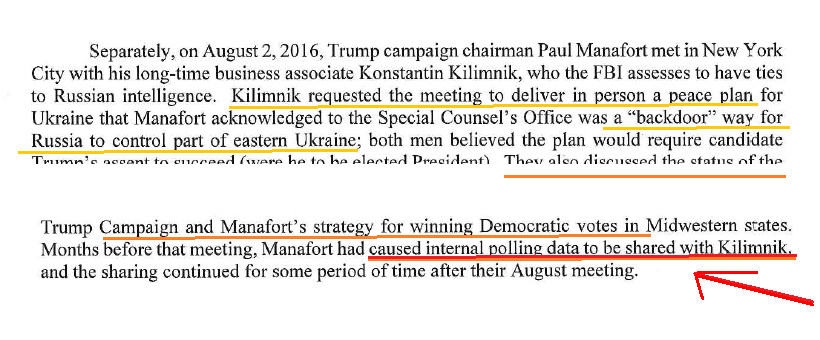The image is a scan or screenshot of two paragraphs of black text on a pure white background. The text is formatted in a standard font, with certain lines underlined in different colors: yellow, orange, and red. The top paragraph begins with the date "August 2, 2016" and details a meeting in New York City between Trump campaign chairman Paul Manafort and his longtime business associate, Konstantin Kilimnik, who the FBI assesses to have ties to Russian intelligence. Notably, the line “Caused internal polling data to be shared with Kilimnik” is prominently underlined in red and highlighted with a red arrow. Additionally, the line mentioning that the peace plan for Ukraine presented by Kilimnik was seen by Manafort as a "backdoor way for Russia to control part of eastern Ukraine" is underlined in yellow. The image captures that the very bottom line of the top paragraph is partially cut off. The second paragraph includes the red underlined line, “Campaign and Manafort strategy for winning Democratic votes in Midwestern states,” and continues to explain how Manafort had shared internal polling data with Kilimnik months before their meeting, with the sharing continuing for some time after.